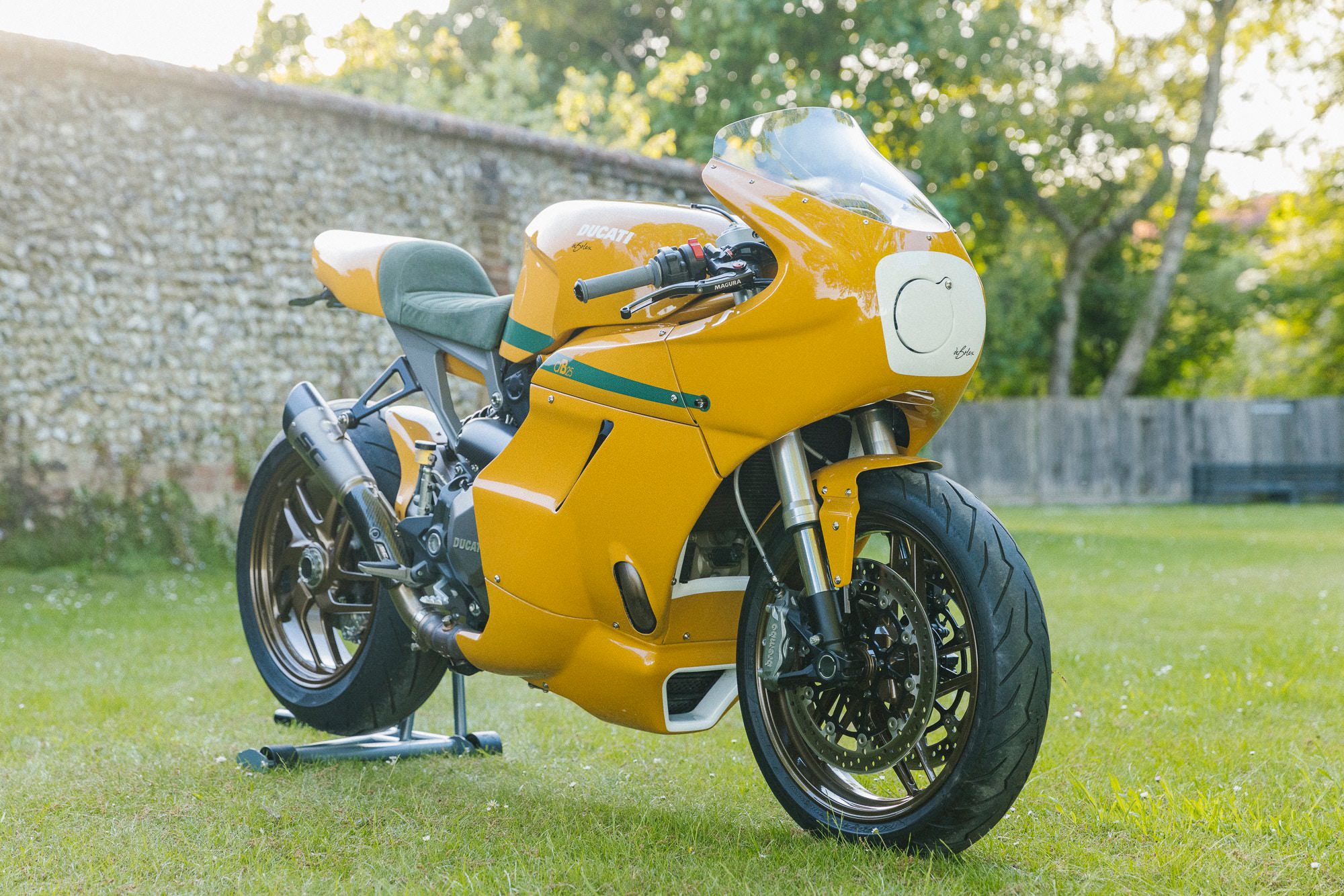A vibrant yellow motorcycle rests elegantly in a lush green grass field. To the left, there stands a grayish brick wall, adding a rustic charm to the background. On the right, a short, dark gray fence is partially hidden by tree trunks, which rise upwards, their branches adorned with abundant green leaves. The motorcycle, facing to the right, features a seat in a light green hue, with a darker green stripe running through its body, adding a touch of contrast. Its front line is protected by a white cover, presumably for safeguarding purposes. The wheels are entirely black, giving the bike a sleek appearance. Attached to the back wheel is a small stand, which elevates the wheel slightly off the ground. This stand features a silverish-white bar, while the part touching the ground is a bright, dark green, illuminated by the sunlight.